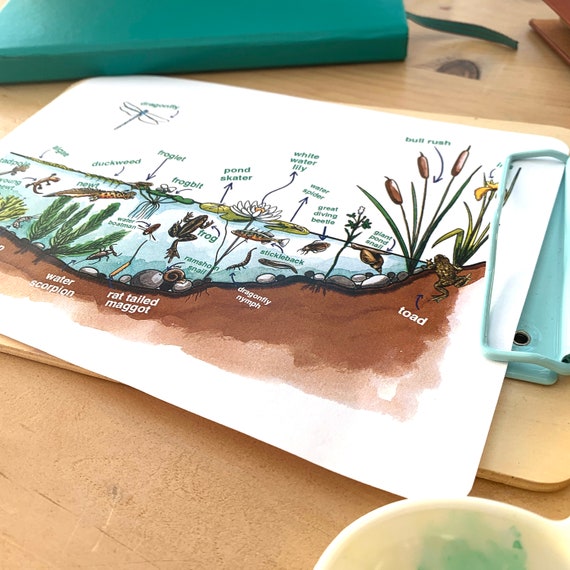The photograph depicts a light blue clipboard with a piece of white paper clipped onto it, resting on a wooden table. The clipboard is positioned with a slight side view of a detailed 2D cross-sectional illustration of a pond and its surrounding ecosystem. Above the clipboard, partially covering the top center and left, is a darker blue book with a visible bookmark on the right side. 

The illustration on the paper portrays a pond with various labeled plant and animal life both in and around the water. Visible in the water are frogs, dragonflies, duckweed, pond skaters, great diving beetles, and giant pond snails among other species. The depiction also includes underwater plants and dirt extending up to the shore on the right side, where a toad is seen alongside a bulrush plant. Detailed labels identify each species in green text, with additional white text providing further descriptions at the bottom. 

In the bottom right corner of the image, partially visible, is a white cup containing green paint, contributing to the scene's artistic setup.